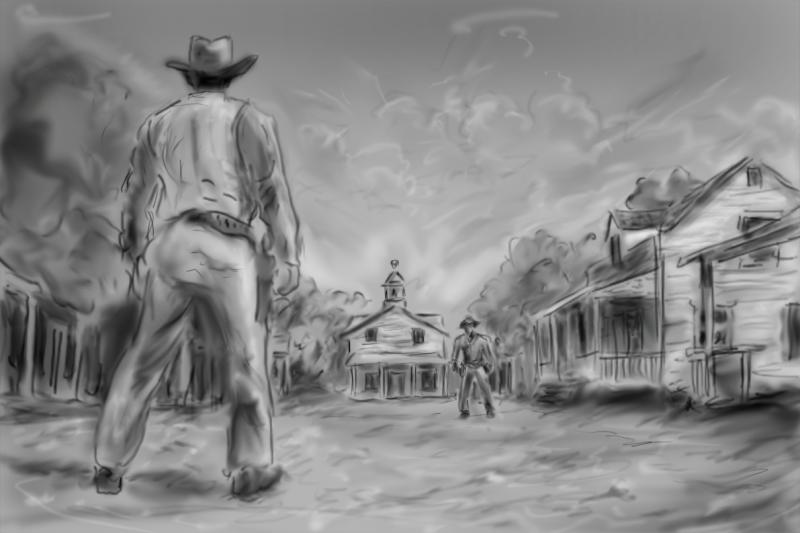This is a vintage-looking grayscale sketch, seemingly drawn in pencil or charcoal, capturing an evocative scene from the U.S. Wild West era. The composition showcases an old Western street lined with homes on the right and a series of buildings, including what might be a saloon or a church, in the distance. The sky is depicted with cloudy, smoky hues, adding to the dramatic ambiance. In the foreground, two cowboys are poised for a standoff. One cowboy, standing to the left, faces away from the viewer, wearing a hat, boots, and a holster with a gun on his right hip. His arms are tense and prepared to draw. On the right, further down the road, the second cowboy stands facing the viewer, similarly dressed and ready for action. The scene is filled with tension, with the sketch’s smudged, blurred lines contributing to a sense of motion and anticipation.